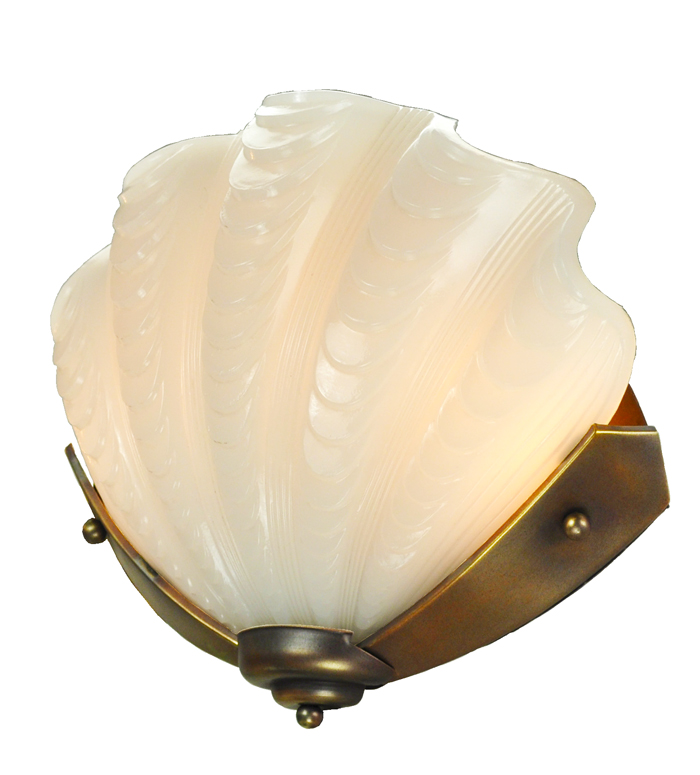This image showcases a meticulously trimmed wall sconce that fills the entire frame without any background or border. The sconce features a prominent shade resembling a scallop shell, characterized by ribbed detailing and a soft, opaque white finish. This elegant shell-shaped shade seamlessly connects to a base made of bronze, which gracefully follows the bottom edges of the shell. Two round screw cap covers are visible on either side of the base, securing it in place. The shell is mounted on a disc-shaped bronze base, which is layered with another disc on top, and concludes with an additional round screw cap cover. This final section houses the light bulb, completing the intricate and classic design of the wall sconce.